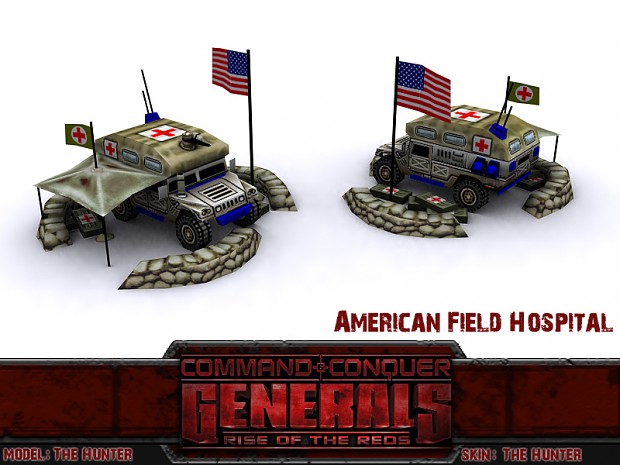The image has a lower banner with red font reading "American Field Hospital," set against a dark grayish-black background, and below it, "Command and Conquer: Generals - Rise of the Reds" is displayed. To the left, the text "Model: The Hunter" and "Skin: The Hunter" is noted. Featured prominently in the image are two computer-generated military vehicles, each adorned with the Red Cross emblem and American flags, indicating their purpose as medical vehicles. One vehicle faces forward, while the other is angled with its front end pointing to the back of the picture. Both vehicles are connected to a tented area, possibly a mobile medical station, and surrounded by a stone-like border. Medical supplies are scattered on the ground near them. The overall scene mimics a realistic American field hospital setup, likely an ad for a game or toy from "Command and Conquer: Generals - Rise of the Reds."